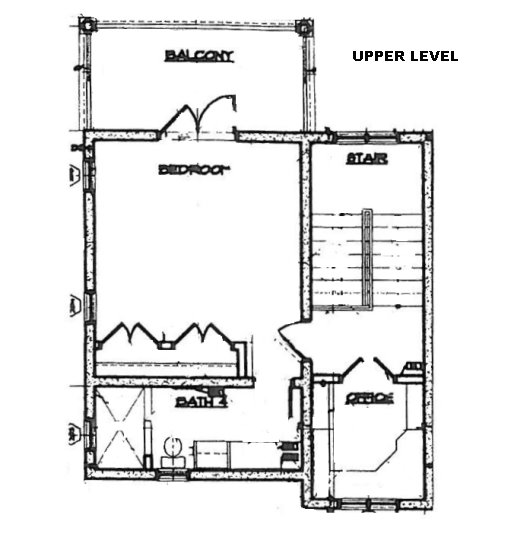The image depicts a black and white, low-resolution floor plan of the upper level of a house. At the top of the diagram, there is a balcony accessible through a door, connected to the main bedroom. The balcony, about half the size of the main bedroom, provides an elevated outdoor area. Opposite the balcony within the bedroom space is a closet featuring double doors for a full view upon opening. Adjacent to the closet, a door leads to an ensuite bathroom equipped with a shower, bathtub, toilet, and sink, offering a comprehensive set of amenities. 

To the right of the bedroom, the main entrance opens to a hallway. Turning left from this entrance leads to a dual-flight staircase descending to the first floor. Heading right, the hallway provides access to two doors leading into an office space. This office room on the upper level includes built-in cabinets, offering ample storage and workspace. Altogether, the floor plan details a well-organized upper level, with distinct areas for relaxation, storage, and work.